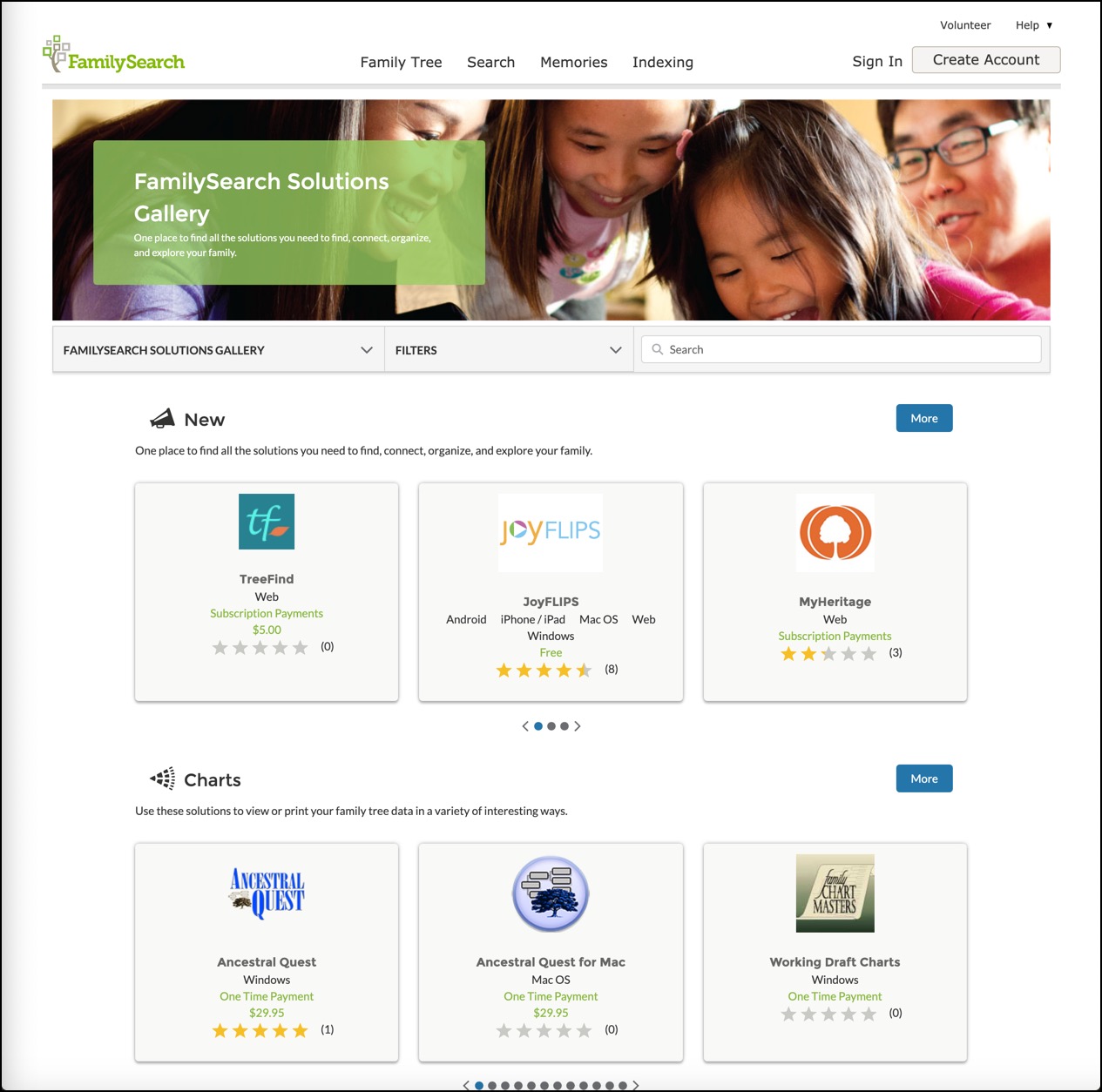Website Screenshot of FamilySearch Solutions Gallery:

The screenshot depicts a square-oriented webpage from FamilySearch with a white background and a thin black border. At the upper left corner, the website name "FamilySearch" is prominently displayed. Adjacent to the top edge of the image are tabs labeled "FamilyTree," "Search," "Memories," and "Indexing." On the upper right-hand side, there is a sign-in box accompanied by "Volunteer" and "Help" buttons.

Directly below this header section, a photographic strip showcases four smiling individuals. A translucent green text box overlay on the left side of this strip reads "FamilySearch Solutions Gallery."

Beneath the photographic strip lies a very light gray banner that reads from left to right, "FamilySearch Solutions Gallery filters." The banner includes a white text search box for user input.

The main content area below the banner consists of six very light gray boxes. At the top of these boxes, a headline reads "New - One place to find all the solutions you need to find, connect, organize, and explore your family." The top row of boxes features labels such as "TreeFindWeb," "JoyFlips," and "MyHeritage," each box accompanied by an icon and a small blue "More" button at the right.

The bottom row contains boxes labeled "AncestralQuest," "AncestralQuest for Mac," "Mac Operating System," and "Working Draft Charts." Each of these boxes also includes icons, text descriptions, and a star rating with the number of reviews.

At the very bottom center of the image, there is a pagination control for navigating through the gallery. This includes several very small gray circles and left and right arrows for scrolling.

Overall, the screenshot provides a comprehensive snapshot of the FamilySearch Solutions Gallery page, highlighting its main features and navigation options.